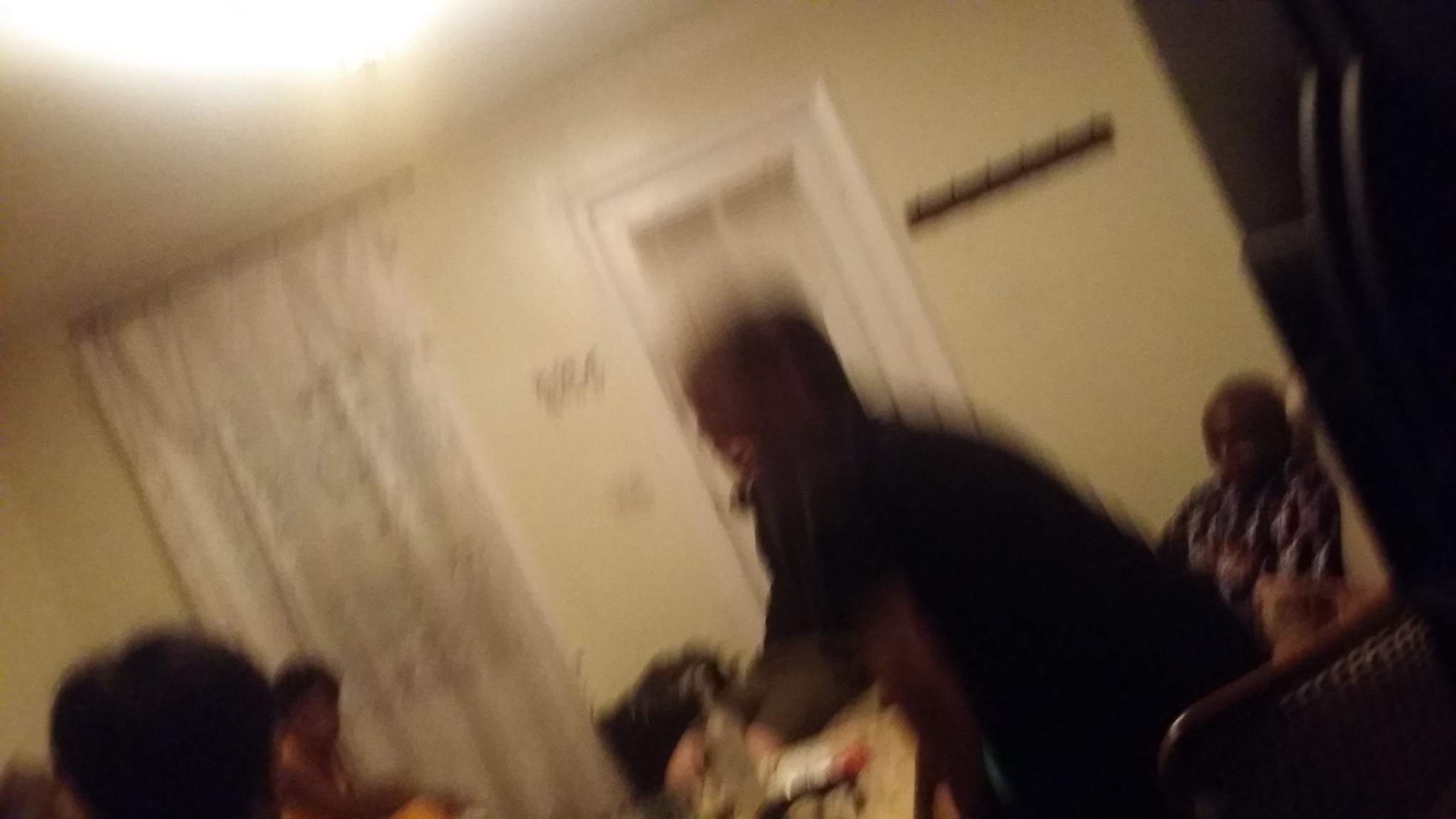This is a vibrant color photograph captured inside a cozy living room, buzzing with life. The image, though slightly blurry, depicts a warm gathering of at least four people, possibly more, comfortably seated in various chairs and on a couch. They are arranged in a circle, engaged in what appears to be an animated conversation. Centrally placed in the room is a long coffee table that adds to the communal setting. 

In the lower right-hand corner of the photo, one individual is standing, seemingly mid-conversation with a person directly across from them. The background reveals a wall with a door and a convenient coat hanger, adorned with hats and coats. To the left, a window draped with a light white curtain allows soft, natural light to seep in, complementing the bright ceiling light that illuminates the entire room. The scene is a snapshot of conviviality and togetherness, capturing a moment of shared stories and connections.